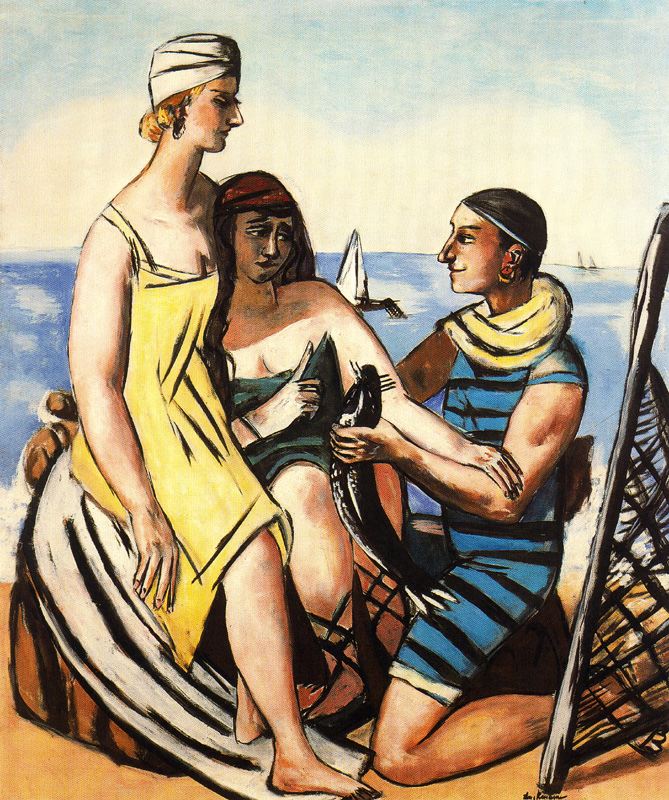The painting depicts a vibrant beach scene featuring three distinct individuals against a backdrop of a cloudy sky and calm ocean. On the right, a man is kneeling on sand, smiling and gazing to the right. He has short dark hair and wears a yellow scarf around his neck, along with a blue swimsuit adorned with black stripes. With a cheerful demeanor, he holds a large dark fish in his left hand, which features notable whiskers. The man's uncovered shoulders enhance his beach-ready appearance.

The central figure is a red-haired woman, who appears anxious with a frightened frown on her face. A shadow partially obscures her expression, extending over her chest. She holds a green towel that partially covers her cleavage, while her right arm rests over the arm of the man holding the fish. Her knees are tucked beneath her, concealed between the man and the other woman seated beside her.

To the far left is the tallest figure, a woman wearing a light sundress that drapes elegantly over her slender frame, revealing some cleavage next to the red-haired woman’s head. She has a white scarf tied like a turban around her head, with blonde hair peeking out beneath it. A long black earring complements her features. Her left arm hangs down, almost reaching her knees.

The trio sits on a structure resembling a stack of wood covered with a white towel, while a fisherman's net lies to the right of the man. In the distance, the serene blue ocean is dotted with small sailboats, blending whites and grays into the waves. The sky above is a mix of hazy white, gray, and hints of blue, adding a dreamy quality to the scenic backdrop.